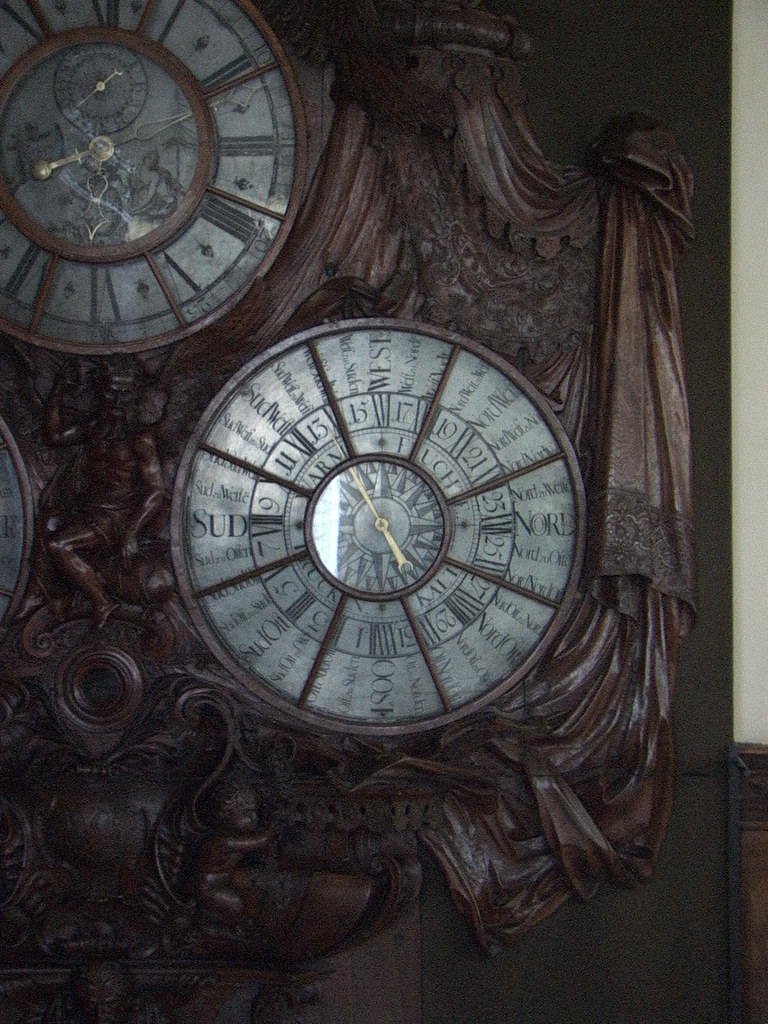This photograph captures an exquisitely detailed clock made from dark chocolate-colored wood. The clock is adorned with an array of intricate carvings, including motifs that resemble the folds and drapery of a Grecian robe, leaves, and floral designs. Prominently featured are two carved figures: a man dressed in what appears to be a toga and a cherubic baby. At the top of this elaborate wooden structure is the clock face, which boasts finely crafted gold hands. Centrally located within the clock face is an additional feature displaying numbers and a day category, suggesting it functions as a date clock as well. The overall craftsmanship and the rich details of these carvings highlight the artistic and historical significance of this timepiece.